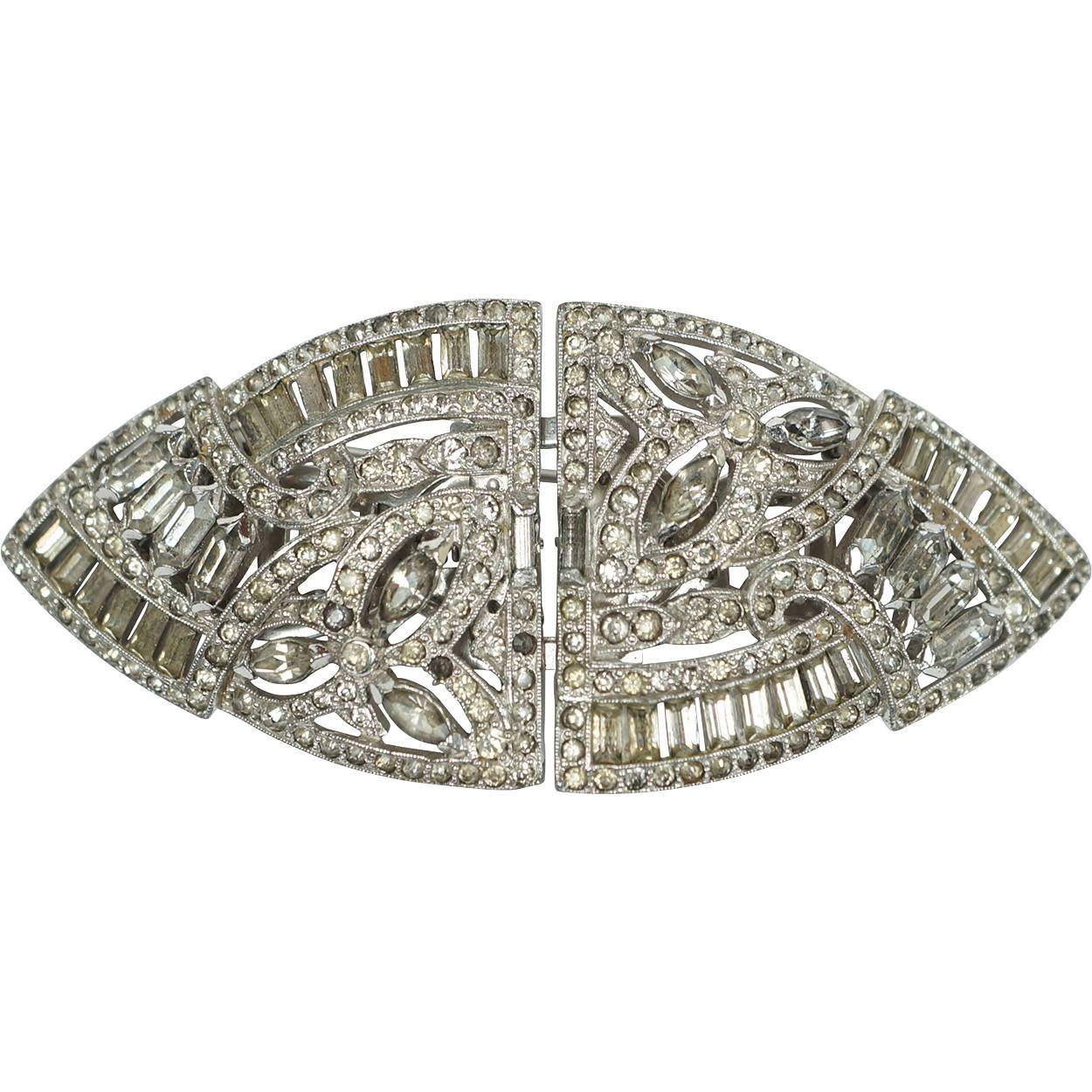The image showcases a piece of vintage costume jewelry that appears to be a silver-colored belt buckle or collar pin set. This accessory is composed of two separable halves, suggesting it can clasp or connect. The design features an ornate, elaborate pattern with ridges and embedded rhinestones of various shapes, including long emerald-cut, marquee (pointed oval), and round. While some rhinestones remain clear and pristine, others have yellowed or are missing. The background is a clean white, highlighting the jewelry's intricate details and numerous crystals that adorn its edges and interior pathways. Despite its age, the piece shows no signs of rust or damage, maintaining a bright and collectible appearance.